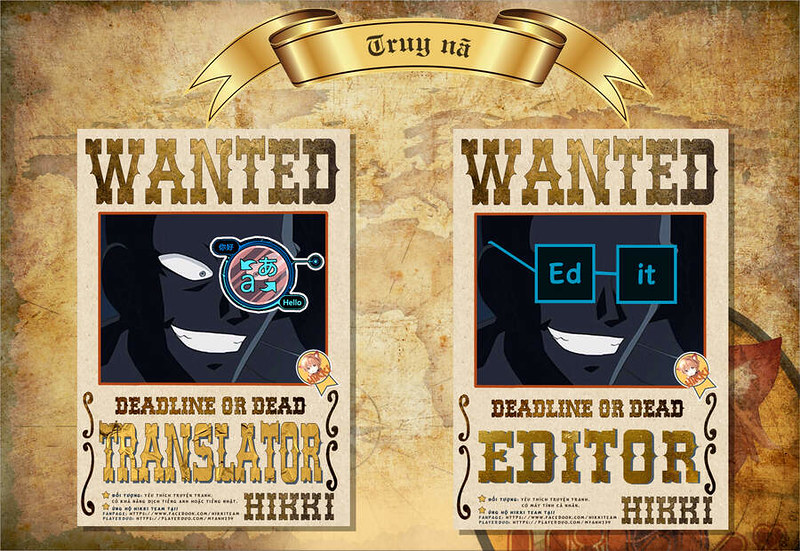The image features a vintage-style recruitment poster set against a weathered, parchment-like background that resembles an old map, complete with a golden ribbon bearing indecipherable text at the top. The centerpiece consists of two Western-style "Wanted: Dead or Alive" posters overlaid with golden lettering that reads "WANTED."

The left poster, labeled "Translator," showcases a dark-skinned figure smiling widely, with a distinctive blue circle covering their left eye. A central round emblem contains various characters, possibly indicating translation capabilities from English to another language like Chinese. The right poster, labeled "Editor," portrays the same figure now adorned with glasses formed by two square frames. The left frame contains "ED" and the right frame "IT," together spelling "EDIT."

Both posters present the enigmatic character in an almost animated, cartoon-like style, set against a cohesive golden background, emphasizing their roles for the desired project.